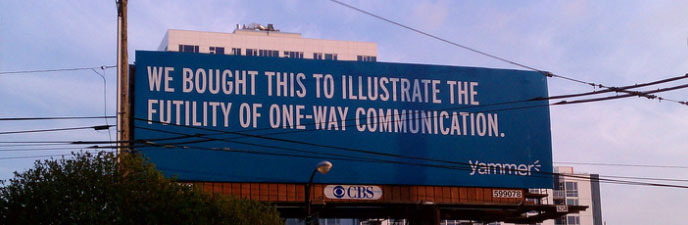This photograph captures a striking outdoor billboard from the company Yammer. Dominating the scene, the billboard features a dark blue background with bold white capital letters reading, "WE BOUGHT THIS TO ILLUSTRATE THE FUTILITY OF ONE-WAY COMMUNICATION." At the bottom corner of the billboard, the Yammer logo is prominently displayed in white. The billboard belongs to CBS, as indicated by a CBS logo on a white oval beneath it. The billboard is positioned amidst a backdrop of a clear, bright blue sky with white and faint gray clouds. It’s flanked by utility wires, with a telephone pole to its left. In the foreground, leafy green branches of a tree partially obscure the view. Behind the billboard, a high-rise apartment building with white walls and numerous windows is visible. An additional detail includes a pink balloon affixed to the billboard, adding a whimsical touch to the scene.